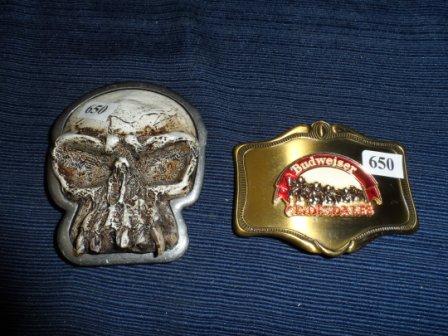This photograph features two small, metal objects placed side by side on a slightly wrinkled blue corduroy fabric background that runs horizontally. On the right is a gold-colored belt buckle-shaped piece, adorned with an enamel print depicting the Budweiser Clydesdales, with a red banner reading "Budweiser" over the Clydesdales and the word "Clydesdales" beneath the line of horses. On the left, the other object is a dull silver-toned metal piece, inset with what appears to be a white skull, either of a gorilla or human, with gray and brown detailing in the eye sockets and mouth. Both objects bear a white sticker with the number 650, indicating they may be for sale or part of a collection.